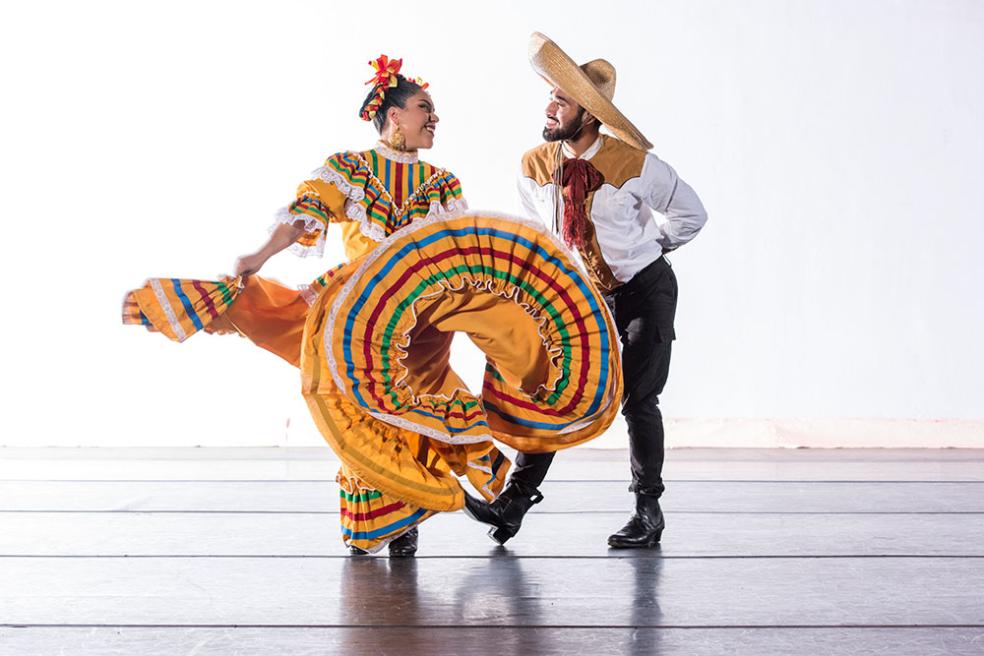This photograph captures a vibrant moment between two dancers, presumably partaking in a Mexican traditional dance on a polished wooden floor. The woman, elegantly dressed in a floor-length, bright yellow dress adorned with white ruffles and multi-colored ribbons in blue, red, and green, is caught in the mesmerizing swirl of her skirt, which she holds up with her right hand. Her ensemble is complemented with a yellow and orange feathered wreath in her hair and large, dangling earrings, all adding to her radiant smile as she gazes at her dance partner. The man, a Hispanic male with a beard and mustache, stands to her right, smiling back at her. He is dressed in a striking white western-style shirt adorned with brown shoulder patches and a tie featuring beige and red accents. His outfit includes dark pants and heeled black leather boots, and is topped off with a traditional, large-brimmed straw sombrero. The pair's infectious joy and colorful attire create a vivid and lively scene against a simple backdrop, highlighting the elegance and spirited nature of their dance.